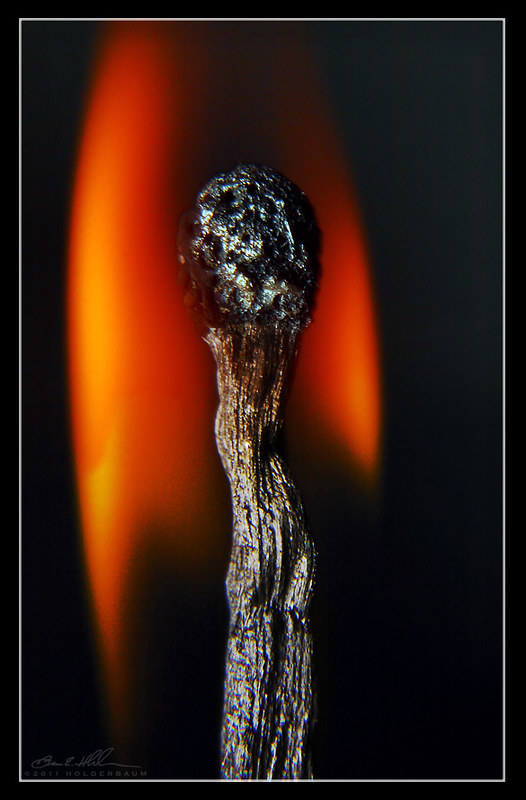The image is an artistic poster featuring a single central object – a highly detailed, close-up view of a lit matchstick. The poster is framed by a white, thin rectangular border that contrasts sharply with the predominant black background. Emerging from the bottom center of the image, the matchstick extends vertically towards the middle, showcasing intricate details of its charred and deformed head. The burnt match head is depicted in varying shades of black and dark brown, transitioning to a more fiery orange and yellow at the top where it is lit. The flames on the match head emanate bright red and orange hues, with the left flame appearing larger than the right. In the bottom left corner, there’s a faint white signature that reads "2011 Holder Bomb," adding an authentic touch to the artwork.